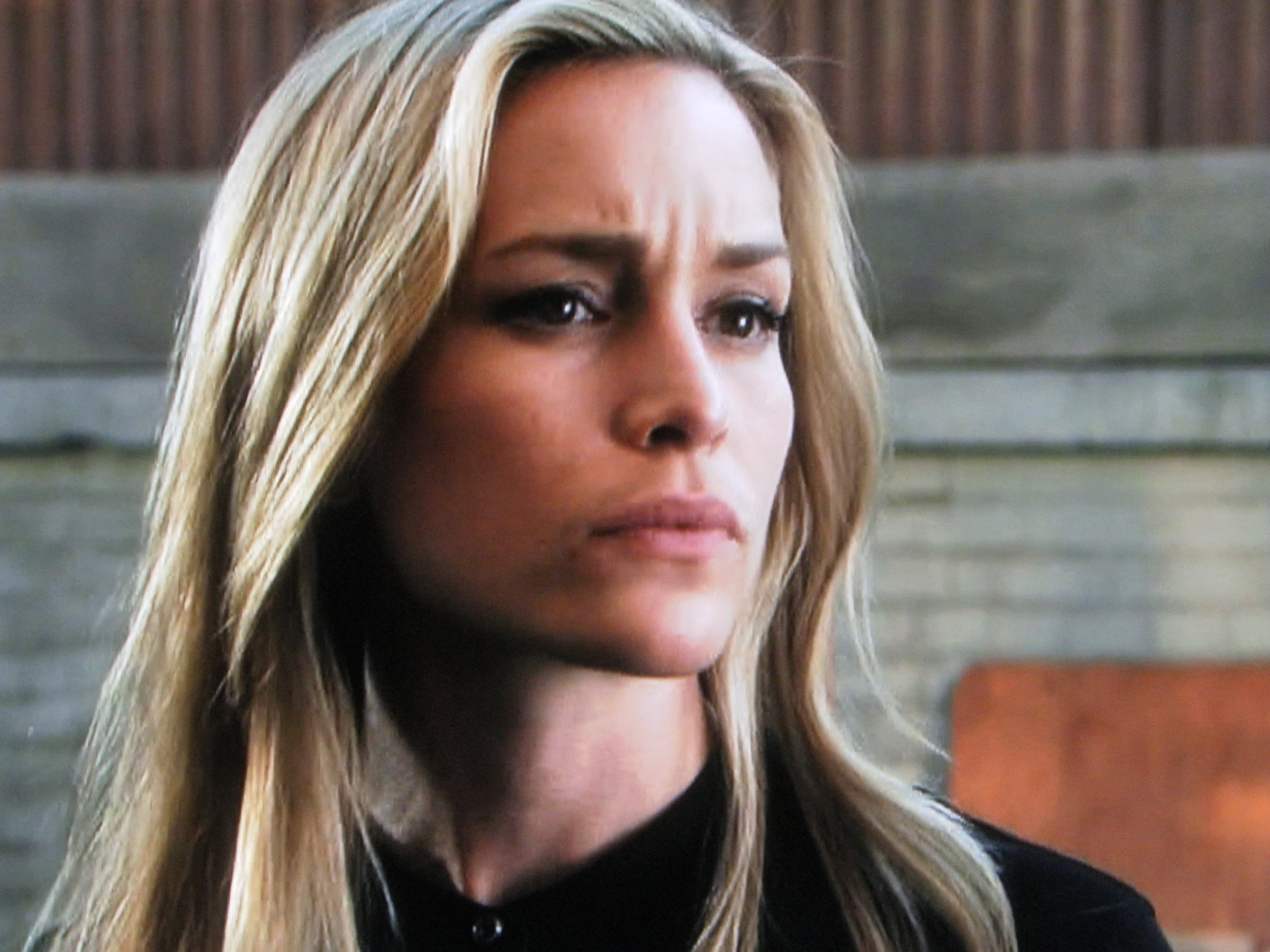The image is a close-up photograph of a young blonde woman, possibly an actress, with light, straight, golden blonde hair that may have some brown accents. Her hair extends beyond her shoulders. She has very dark chocolate brown eyes, and her eyebrows are thin and furrowed at the center, giving her a concerned or serious expression. Her mouth is closed tightly, and her jaw is set, indicating she might be listening intently or examining someone off-frame to her right. She is dressed in a black shirt, and only the upper part of her chest is visible, along with the tip of her right shoulder. The background features a mix of textures: a stone or brick wall with vertical metal poles at the top. There appears to be some wooden planks leaning against the wall, giving the impression of an industrial or possibly outdoor construction site. Overall, the scene looks like a still shot from a film or TV show, capturing a tense or serious moment.